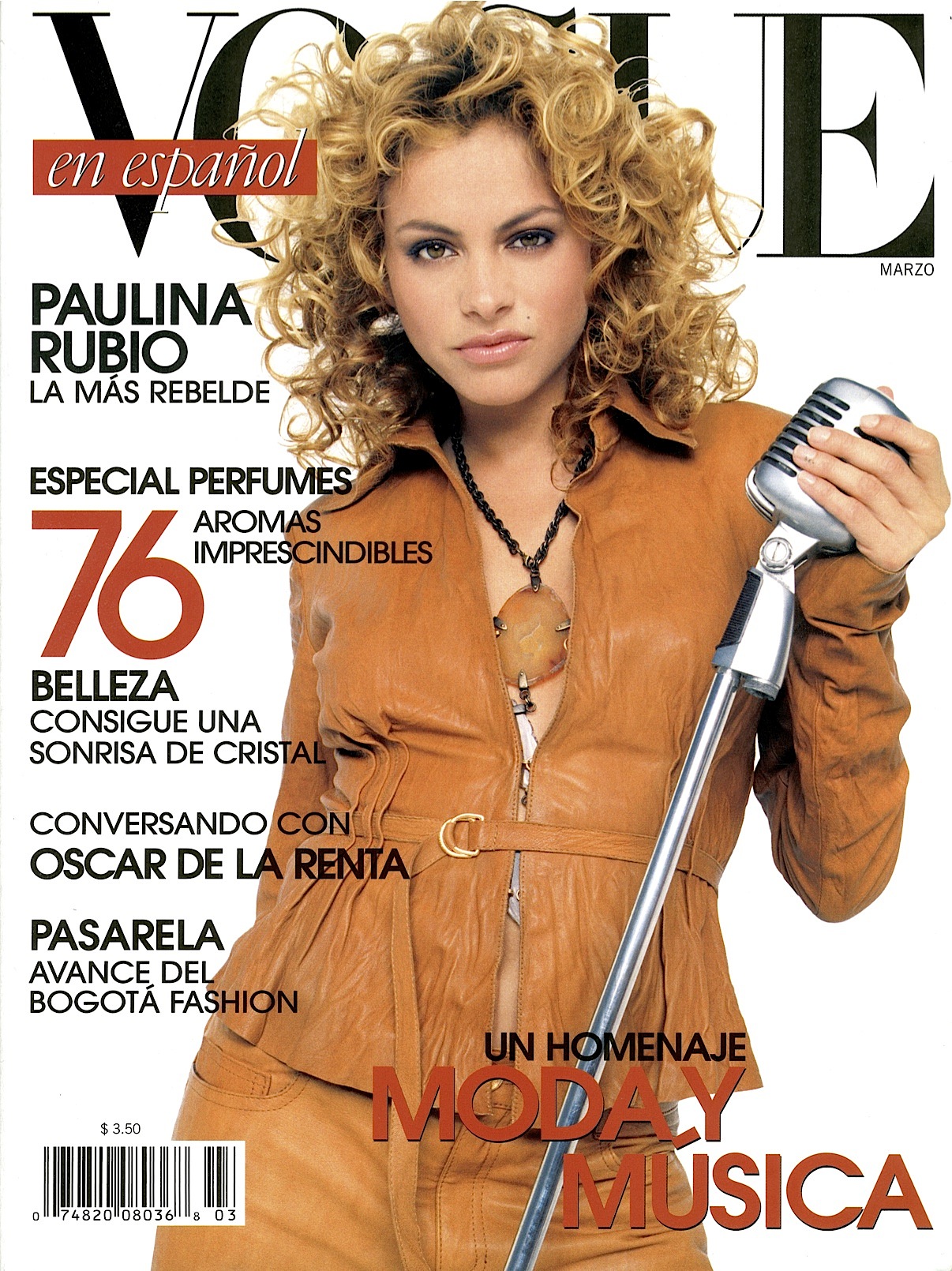On the magazine cover of Vogue en Español, dated for March, the headline reads "Vogue" across the top, partially obscured by the blonde-haired woman’s head. She gazes directly into the camera, holding a silver microphone with a square top in her left hand. The woman is dressed in stylish brown leather pants and a matching long-sleeve jacket, complemented by a corded necklace with an oval-shaped brown pendant. Numerous lines of text decorate the cover, prominently featuring the name Paulina Rubio and phrases such as "Llamas Rebetel", "Especial Perfumes", "76 Aromas Imprescindibles", "Belleza consí una sonrisa de cristal conversando con Oscar de la Renta," and more, suggesting articles inside the magazine. The bottom left corner displays a barcode priced at $3.50 with the numbered sequence 748200803603.